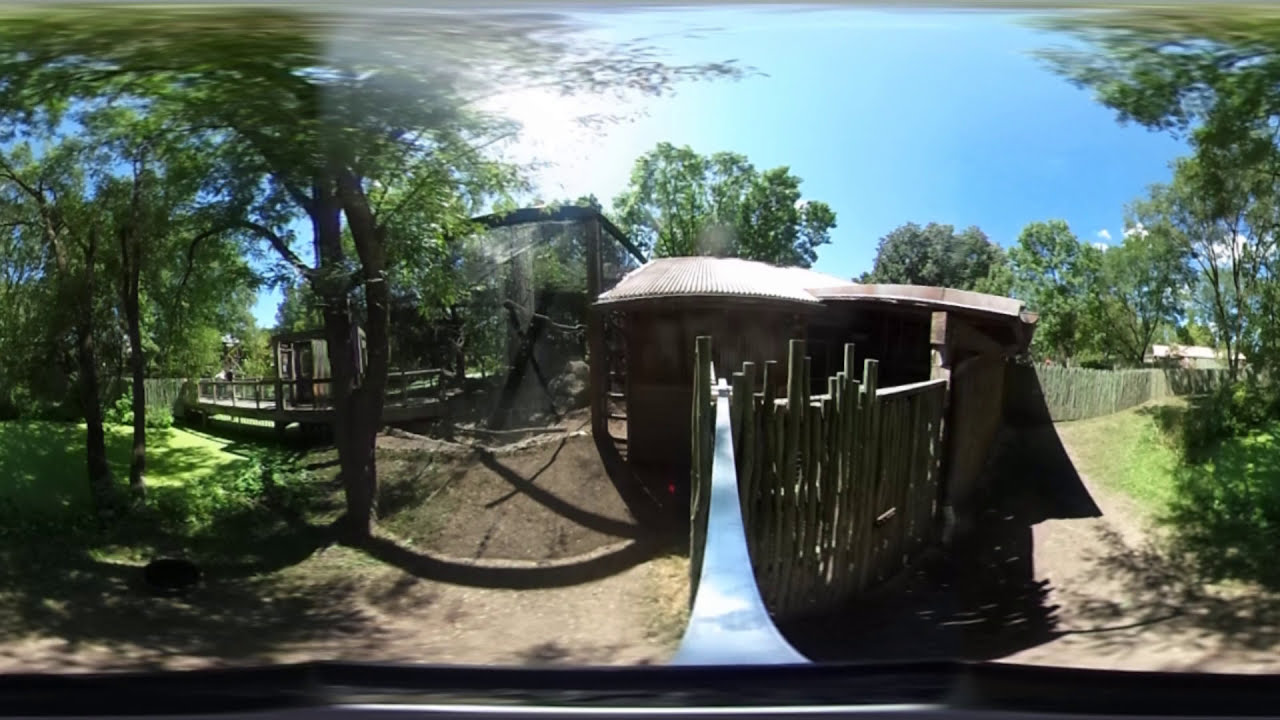The image depicts a rustic, outdoor scene featuring an old wooden structure that serves as both a gate and a door, reinforced by a silver bar across the middle. The structure is built from wooden posts and is accompanied by a shiny roof. To the left, the ground is a mix of gray and beige dirt, leading up to a prominent tree with lush green leaves. Behind the tree is a brown building with a balcony. The central focus is a small, worn-down shack, likely used for animals, which is separated from the road by a wooden fence.

This road, a visible dirt path, extends towards the house, further enclosed by a tall wire fence and an adjacent stone fence on the right. The entire area is surrounded by trees with dense green foliage, framing the house on all sides. The sky is a stunning, clear blue with the bright Sun emitting strong rays, particularly illuminating the left side of the scene. The foreground includes patches of grass and additional dirt paths, blending into the scenic countryside setting.